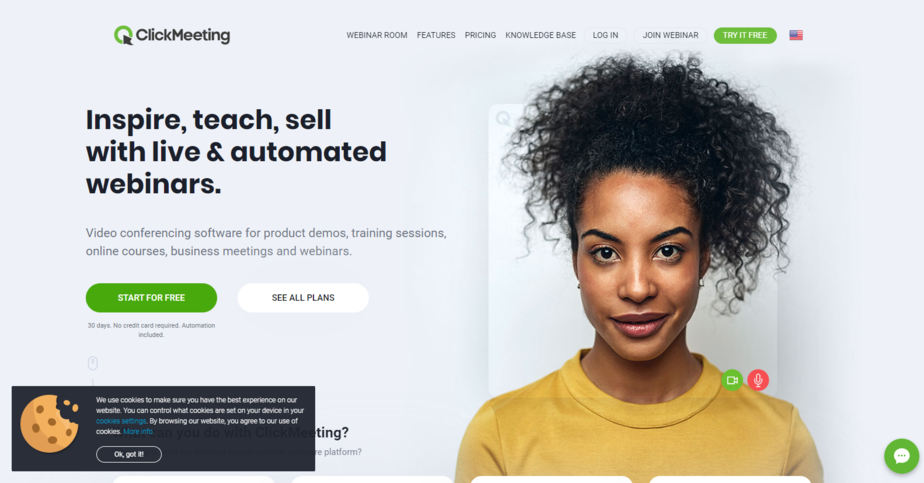This is a promotional image from the company ClickMeeting. At the top of the image, there is a navigation bar with various categories: "Webinar Room," "Features," "Pricing," "Knowledge Base," "Log In," "Join Webinar," and "Try It Free." The "Try It Free" option is highlighted in a green rectangular button. An American flag icon is also present, indicating language or regional settings.

Below the navigation bar, the main header reads, "Inspire, teach, sell with live and automated webinars." A subheader elaborates, "Video conferencing software for product demos, training sessions, online courses, business meetings, and webinars." There are two prominent buttons beneath this text: a green rectangle labeled "Start for Free" and a white rectangle that says "See All Plans." Some smaller print appears under these buttons, likely offering additional information or terms of service.

At the bottom of the image, there is a rectangular area featuring a cookie icon, likely related to the website's cookie policy.

On the right side of the image, an African-American woman is smiling directly at the camera. She is wearing a mustard yellow shirt and her curly black hair is styled in a ponytail. She is also wearing earrings. Near her are a few icons, and there is a speech bubble at the bottom, suggesting interaction or communication features.

Overall, this image encapsulates the user-friendly and feature-rich interface of ClickMeeting, promoting its capabilities for webinars and other online engagements.